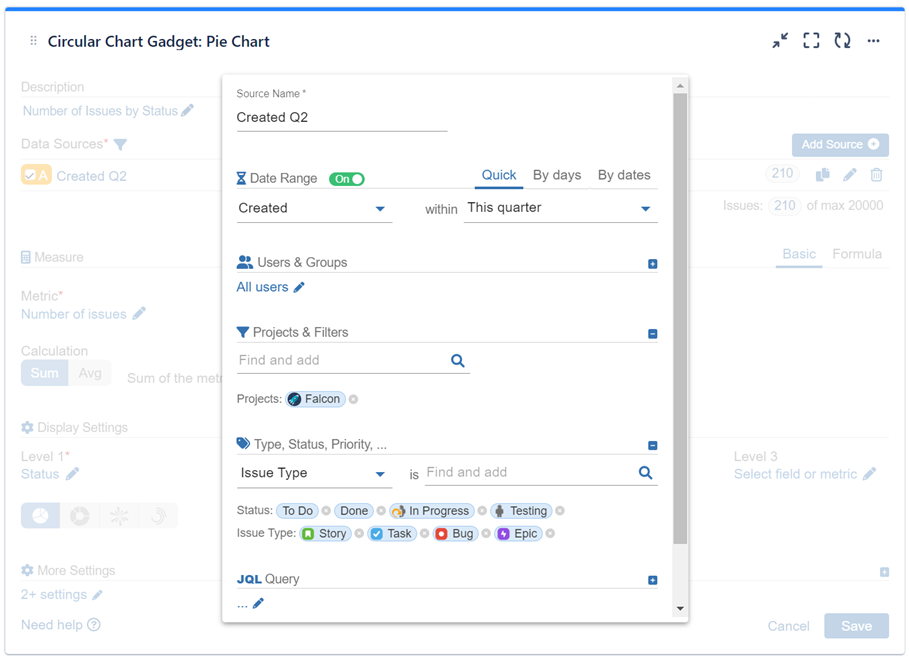This screenshot captures a detailed view of a circular pie chart gadget, created in Q2, set within a project management dashboard. The date range is activated and set to "This Quarter" using the "Quick" option. A dropdown menu allows selection by days or dates. 

At the top, there are sections for "Users and Groups," currently showing "All Users" with an edit option, and "Project and Filters," which includes a search bar to find and add specific projects or filters. The tag “Falcon” is displayed, indicating the project currently viewed.

Below, there's a detailed segment titled "Price Tag," listing type, status, and priority. A dropdown menu under “Issue Type” provides options like story, task, bug, and epic. The status options include “To Do,” “Done,” “In Progress,” and “Testing.” The segment also provides a field to input JQL queries for advanced searching.

In the background, additional interface elements are visible, featuring metric calculations by sum or average, display status, and settings labeled as "Level One." Furthermore, advanced settings options are present. The chart represents 210 issues out of a maximum capacity of 20,000 on a simplistic white background, enhancing readability and focus on the data presented.